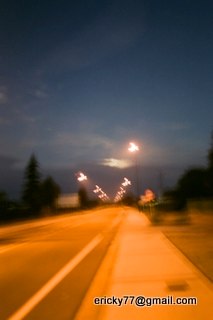A nightly scene unfolds on a dimly-lit sidewalk that glows with a soft, orange-brown illumination. The path is flanked by a series of lampposts, each crowned with a light that casts a gentle glow, stretching endlessly forward into the distance. The posts stand in a rhythm of left, right, left, right, creating a pattern that guides the eye down the length of the road. On either side of the sidewalk, dark silhouettes of trees add a sense of depth and contrast to the scene. Above, a dark sky is scattered with clouds, barely visible against the shadows of the night. The sidewalk itself is a dark gray, marked with white lines that add texture and direction to the path ahead.